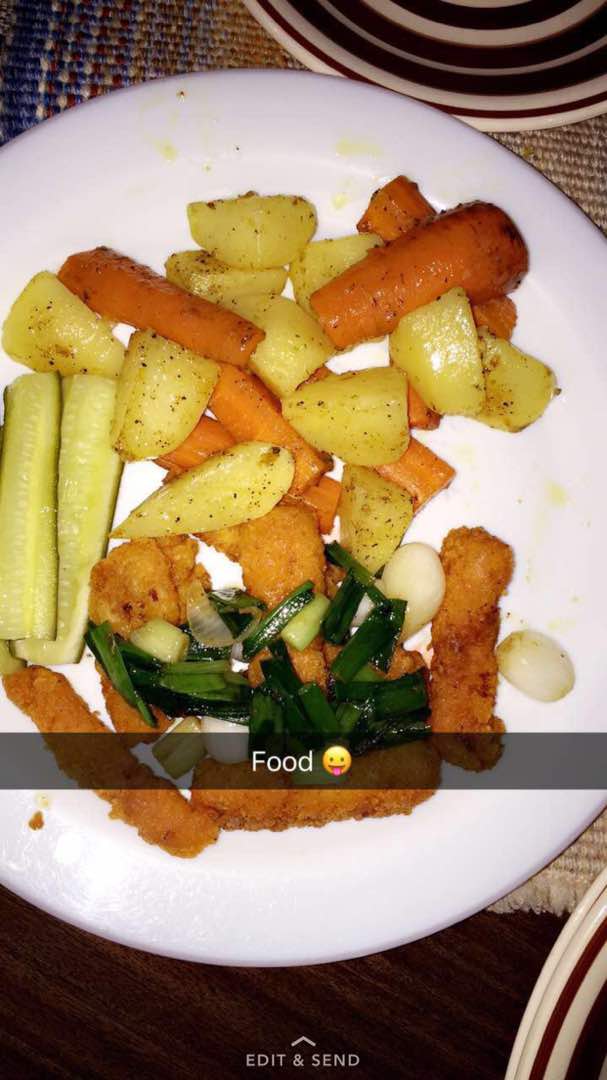This tall, rectangular photograph appears to have been taken on Snapchat. The image, approximately six inches tall and three inches wide, provides a bird's-eye view of a dark brown wooden table set with woven, tan placemats interlaced with blue and red strings. Central to the photo is a bright white plate, extending off both the left and right edges of the frame. Pictured on the plate are roasted strips of carrots, cooked potatoes, possible fried potato-based items like tater tots or chicken fries, two pieces of squash, and a garnish of greens. Additionally, slices of pickles and white onions are visible, suggesting a varied assortment of vegetables. In the bottom portion, horizontally crossing the plate, is a gray bar reading "food" in white font, accompanied by an emoji with its tongue out. The corners of two additional plates appear in the top and bottom right of the image, each featuring white, blue, and dark red stripes. At the bottom center of the image, there is text that reads "edit and send" with an upward arrow pointing towards the lower right corner.